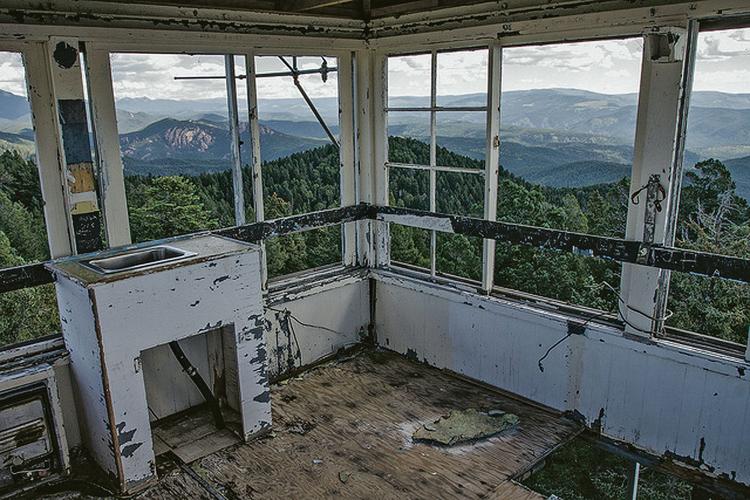The photograph depicts a severely neglected fire lookout station perched on a mountaintop. The interior is dilapidated, with large, open windows on both visible walls, remnants of what once contained glass panes. Where the right and left walls meet, the bottom portion shows a white surface marred by mold and peeling paint. The floor is covered with worn-out, discolored brown linoleum, and to the left, a solitary cabinet with a steel sink, absent its faucet and water source, remains intact despite evident vandalism. Electrical wires dangle from the walls, indicating fixtures that have been ripped out. The view through the empty window frames is breathtaking: a series of mountainous ranges covered in dense, green evergreens transition into steel-gray hues as they recede into the horizon, beneath a sky of white and light gray clouds. The stark contrast between the rundown interior and the pristine, endless mountain scenery highlights the abandonment and decay of what was once an important vantage point for fire rangers.